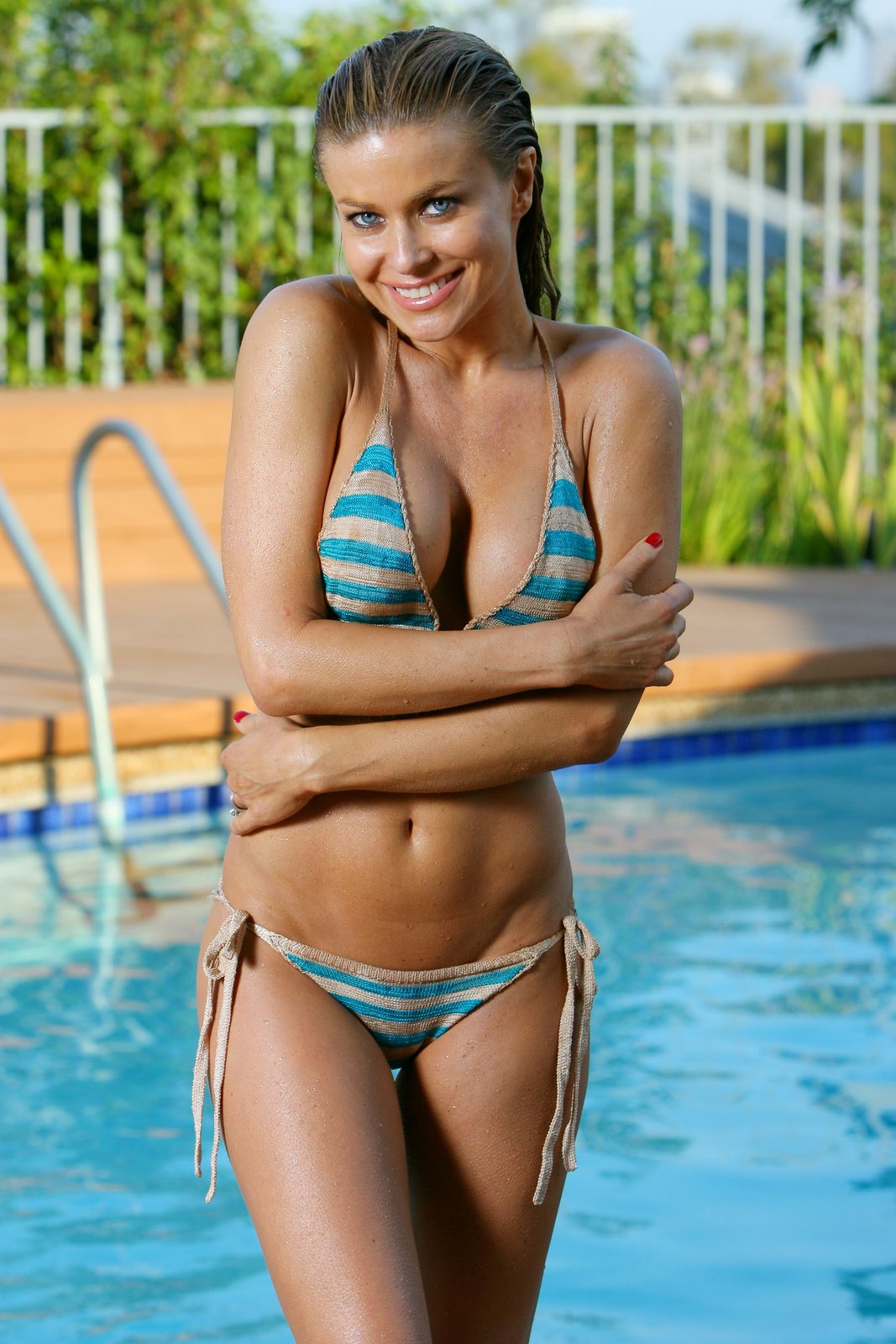In this photo, a woman, identified as Carmen Electra, stands by a pool. She is smiling warmly at the camera, her head slightly tilted, showcasing her light blue eyes and her teeth. Carmen's slicked-back, wet, short brown hair further suggests she has just emerged from the pool, as does her wet skin. She is wearing a striped bikini featuring alternating aqua and beige colors. The bikini top and bottoms are tied with straps that hang down across her otherwise bare legs. Her red-painted nails and a ring on her right hand are visible as her arms wrap around her midsection, giving the impression she might be cold. The background of the image includes a blurry view of the pool, a sidewalk, patches of greenery, a white fence, and some buildings in the distance. Additionally, the pool's blue water and its stair railings are visible on the left side of the photograph, with the sky peeking through in the top right corner.